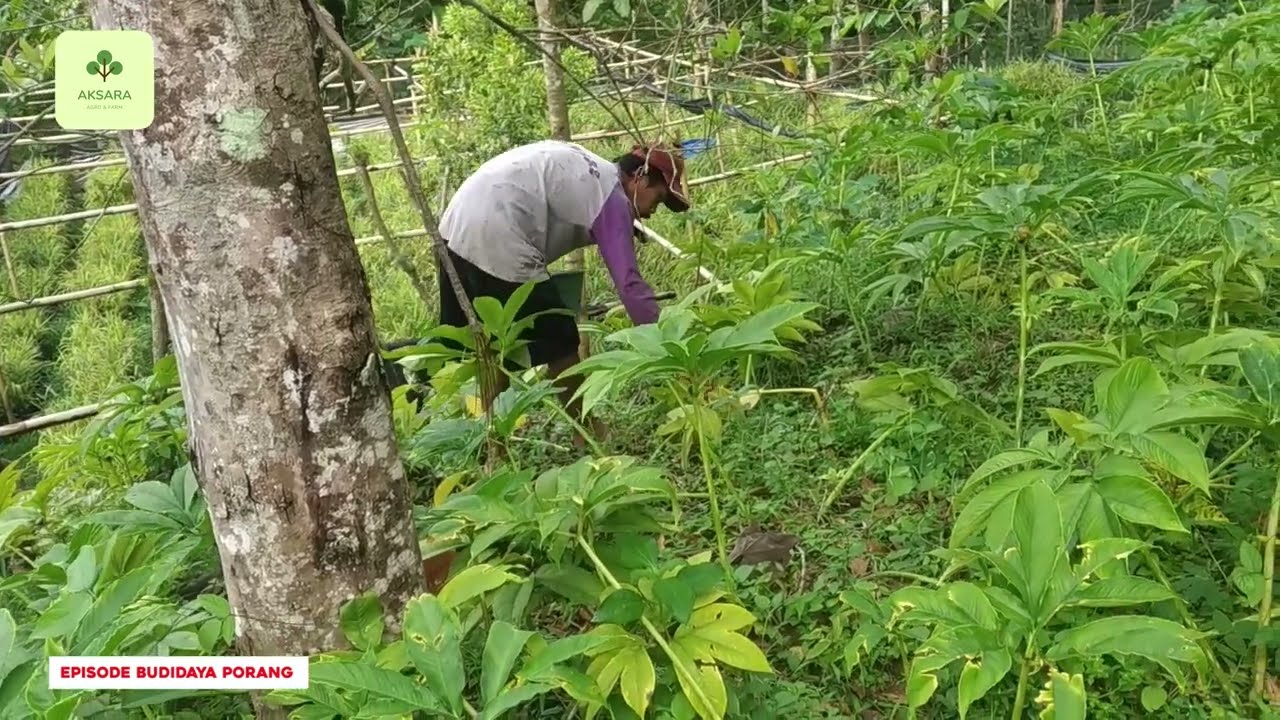The photograph captures an Asian farmer diligently working in a lush, green field under the daylight. He is dressed in a white and purple long-sleeve jersey-style shirt and black shorts, complemented by a brown hat. The man is hunched over, plucking at some tall, thick green plants, potentially flowers or crops. Behind him, a bamboo fence pens a section of the area, adding to the rustic farm setting. A substantial tree trunk is visible on the left side of the image, anchoring the scene. In the lower left corner, a white banner with red text reads "Episode Budidaya Borang," while the upper left corner showcases a light green box featuring the word "Aksara" in dark green font and accompanied by a small icon of a tree. This scene suggests a serene, agricultural environment likely set in an Asian country such as Indonesia, Thailand, or the Philippines.